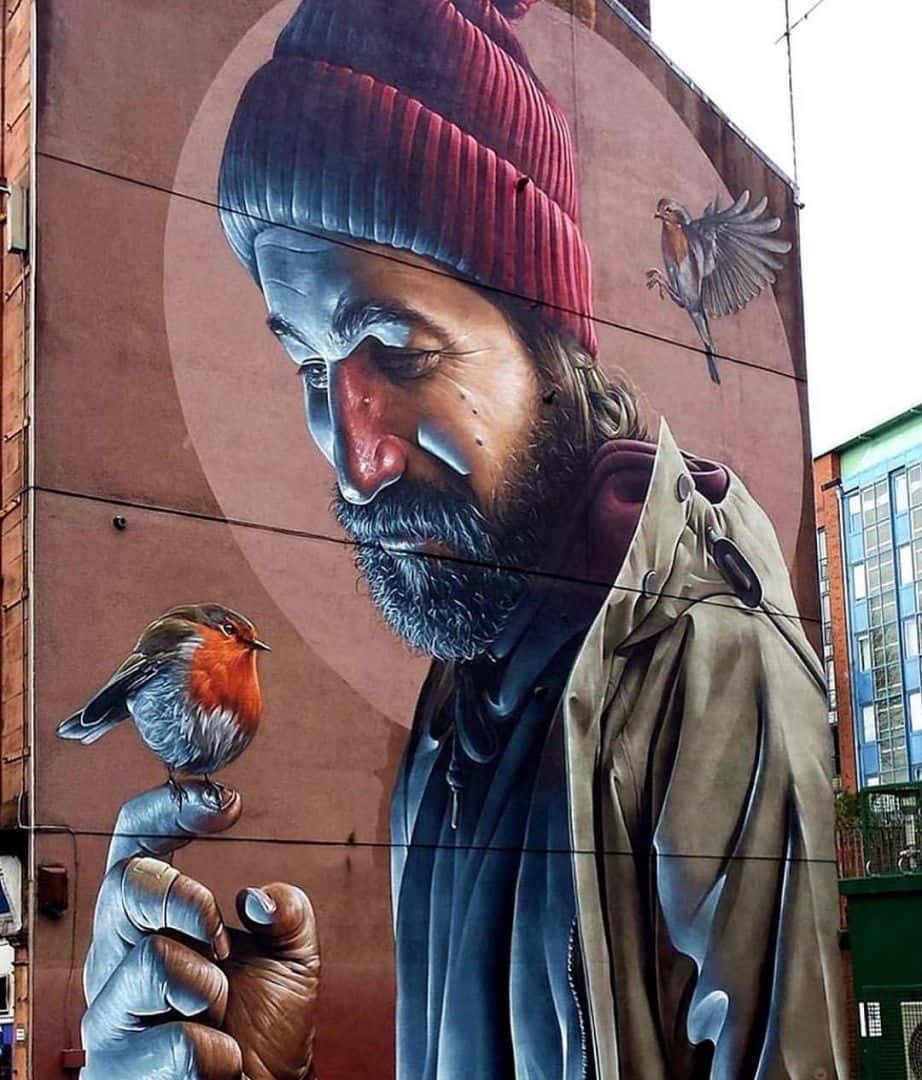The image is an outdoor color photograph taken at street level during daylight, depicting a vivid mural painted on the side of a three-story building. The mural features a detailed, three-quarter view of a bearded man, who appears to be around 35 years old. He is a white male, wearing a red knit cap, a green hoodie underneath a tan hooded jacket, and a blue shirt. The man is looking down at his right hand, which he holds up in front of his face.

Adorning his index finger is a bird, characterized by its red breast, short beak, brown crown, and black feathers. A bandage is visibly wrapped around the middle finger of the man's hand. There is a second bird, hawk-like and with extended talons, flying behind the man's shoulders as if it is about to land on him.

The background of the mural is a rich reddish-brown color, and behind the man's head is a prominent pinkish circle, giving the impression of a halo. The entire scene on this windowless side of the building adds a striking visual element to the urban landscape, drawing attention to its intricate and expressive details.